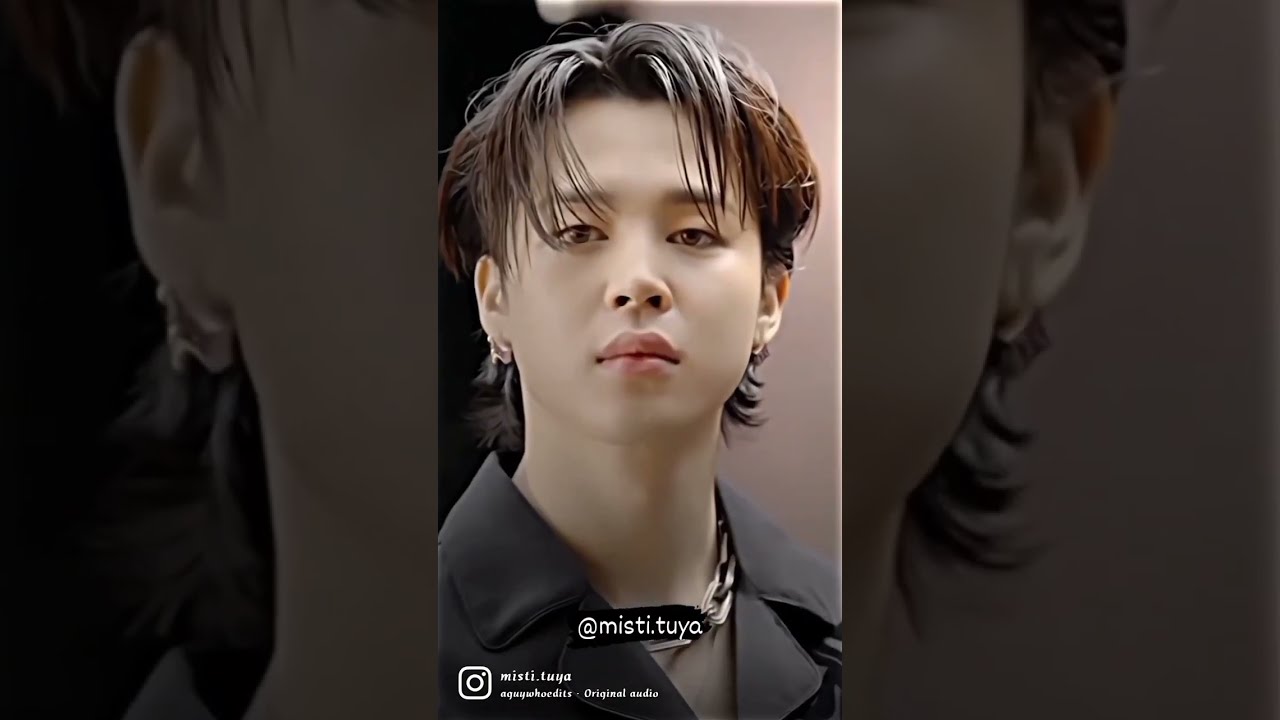This full color photographic image, digitally enhanced and formatted for Instagram, features a striking portrait of a young Asian individual named Misty, with the handle @misty.tuya prominently displayed. Laid out in a horizontally rectangular triptych, the central panel overlays the identical side panels, creating a cohesive tripartite effect. Misty gazes directly into the camera with short, dark hair that falls in a shaggy, eye-covering style, showcasing a smooth, makeup-free complexion. She pairs her look with earrings in each ear and a distinctive silver chain link necklace, complementing her chic black collared top. The left-hand corner of the image also features the Instagram symbol, further indicating its social media orientation.